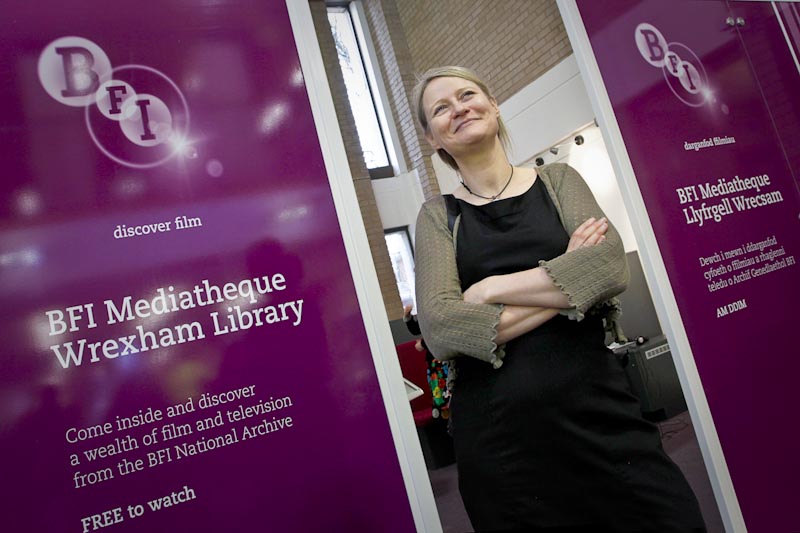In the center of the image, a blonde woman stands with her arms crossed, wearing a grey sweater with three-quarter sleeves over a black full-length dress. A necklace adorns her neck, and she gazes slightly upward with a pleasant expression. The setting appears to be indoors during the day, likely inside a library. Behind her, partially obstructed by her presence, is a door with signs on either side that read: "Discover Film, BFI, Mediatheque, Wrexham Library. Come inside and discover a wealth of film and television from the BFI National Archive, free to watch." Surrounding the woman and the door are various colors, including purple, white, pink, black, gray, blue, yellow, red, and maroon.